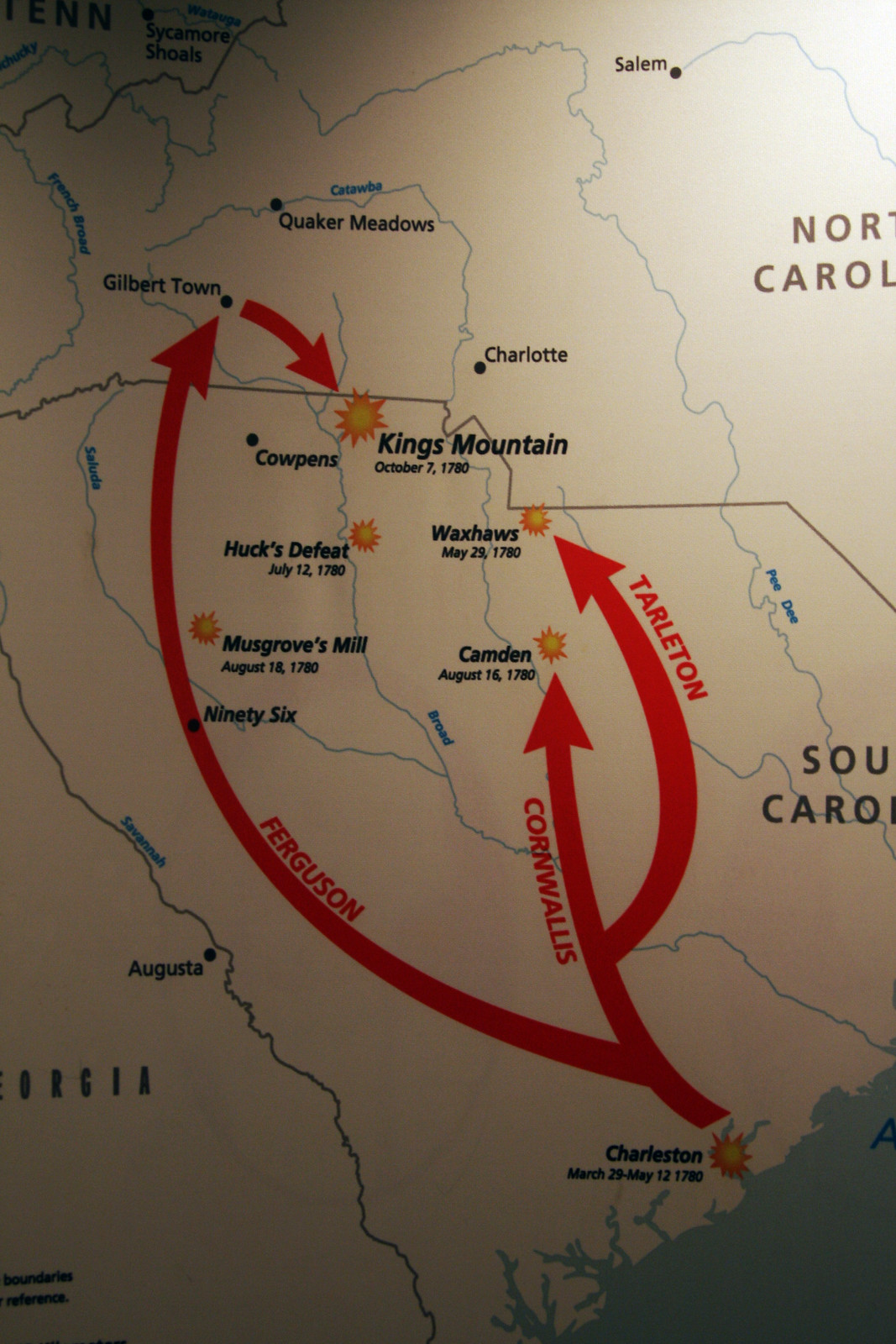This is a vertically aligned rectangular photograph of a historical map, primarily displaying the states of South Carolina, with portions of North Carolina and Georgia also visible. The image is well-lit in the upper right corner but becomes progressively darker toward the bottom left, suggesting it might be mounted on a wall with uneven lighting. The map focuses on significant movements during a military campaign, featuring arrows that represent the paths of three key figures: Cornwallis, Tarleton, and Ferguson. 

Starting at Charleston, marked by an image of a sun, the first arrow curves to the left towards Gilbert Town, North Carolina. The second arrow traces a path up the center to Camden, marked by another sun image, with a branch leading further up and to the left to Waxhaws, also adorned by a sun symbol. The third arrow, representing Ferguson's route, travels past various locations including Musgrove's Mill, 96, Huck's Defeat, and Cowpens, before reaching Gilbert Town and then curving down towards Kings Mountain in South Carolina. Additionally, the map contains textual details, such as dates and names of places, contributing to its informative histographic nature. The top-right corner clearly displays "North Carolina," although part of it is cut off by the edge of the image, with "South Carolina" located below it.